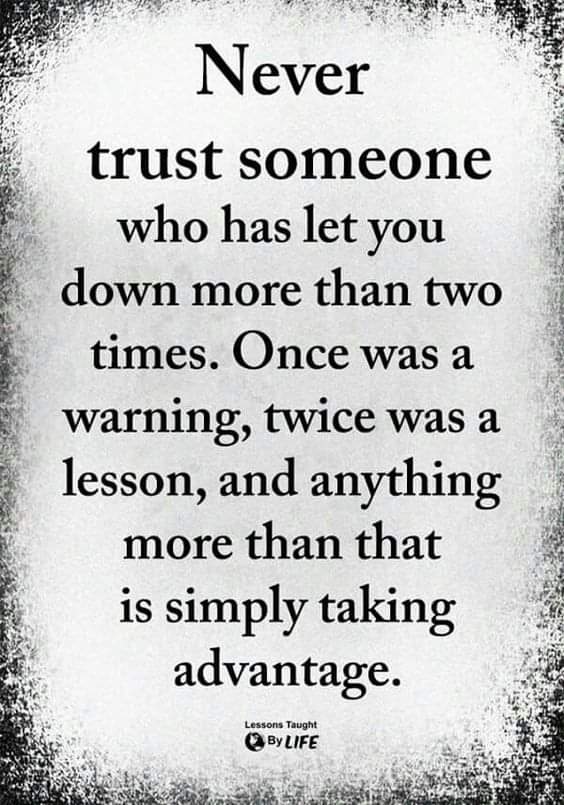The image features an inspirational meme with a predominantly white background that fades into black and gray at the four corners. The text, which is centered and bold black, covers the majority of the image, conveying the message: "Never trust someone who has let you down more than two times. Once was a warning, twice was a lesson, and anything more than that is simply taking advantage." Below this larger text, in much smaller writing, it says, "Lessons taught by life."